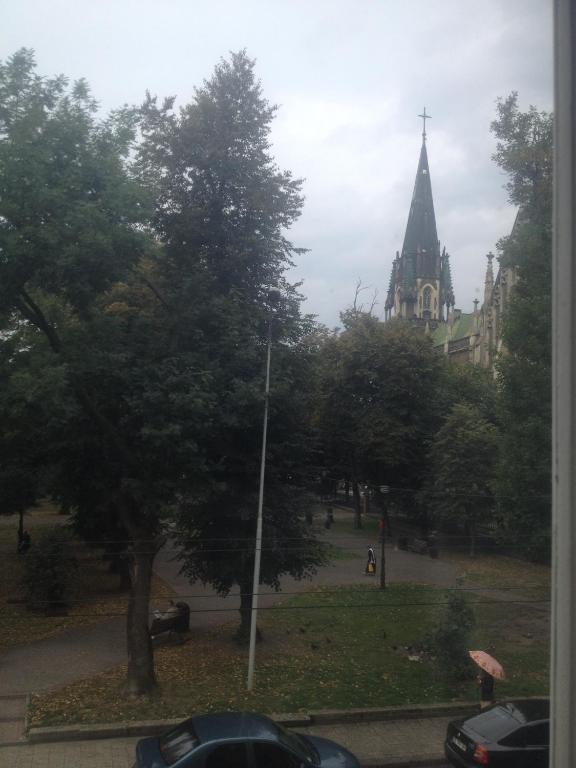This image, likely taken from a higher vantage point such as an apartment or hotel room on at least the second floor, captures a street view transitioning into a quaint park setting. Dominating the scene is an old, intricately designed gothic-style church tower with a cross at the top, rising majestically behind an array of tall trees in the park. The trees, a mix of coniferous and deciduous species, frame the park beautifully. The asphalt walkways within the park are active with several people; one individual carrying a yellow umbrella meanders past a maroon sedan, while another person with a yellow bag walks nearby. Seated individuals occupy benches, adding to the park's serene ambiance despite the cloudy, rainy weather evident from the white-overcast sky. In the foreground, two parked cars, a blue sedan and a partially visible black car, mark the boundary between the street and the park's lush greenery.